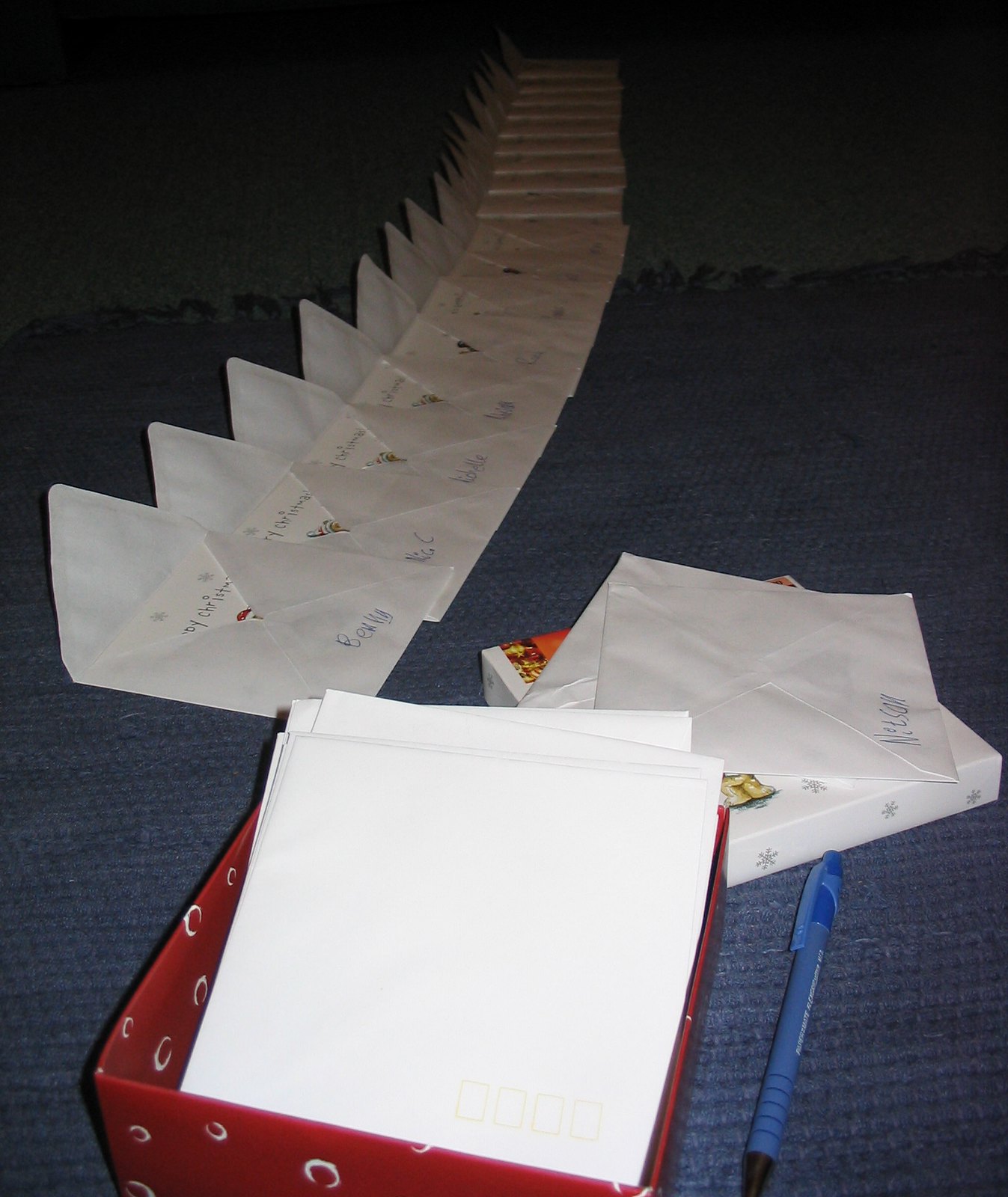This photograph captures a festive and organized holiday card preparation scene. In the bottom left corner, there's a red box adorned with white circle patterns, filled with white envelopes, their tops neatly facing up. Adjacent to the box rests a blue ink pen. Slightly above, a white box decorated with silver snowflakes holds a card-filled envelope with visible writing on the outside. Dominating the upper half of the image, a line of open envelopes, each with a card inside, stretches across the room, fanned out with unsealed flaps pointing upwards. Some envelopes are inscribed with recipient names, such as "Benny," though most names are not legible. The entire setup is laid out on a blue carpet, evoking a sense of a thoughtful and methodical approach to sending out Christmas greetings.